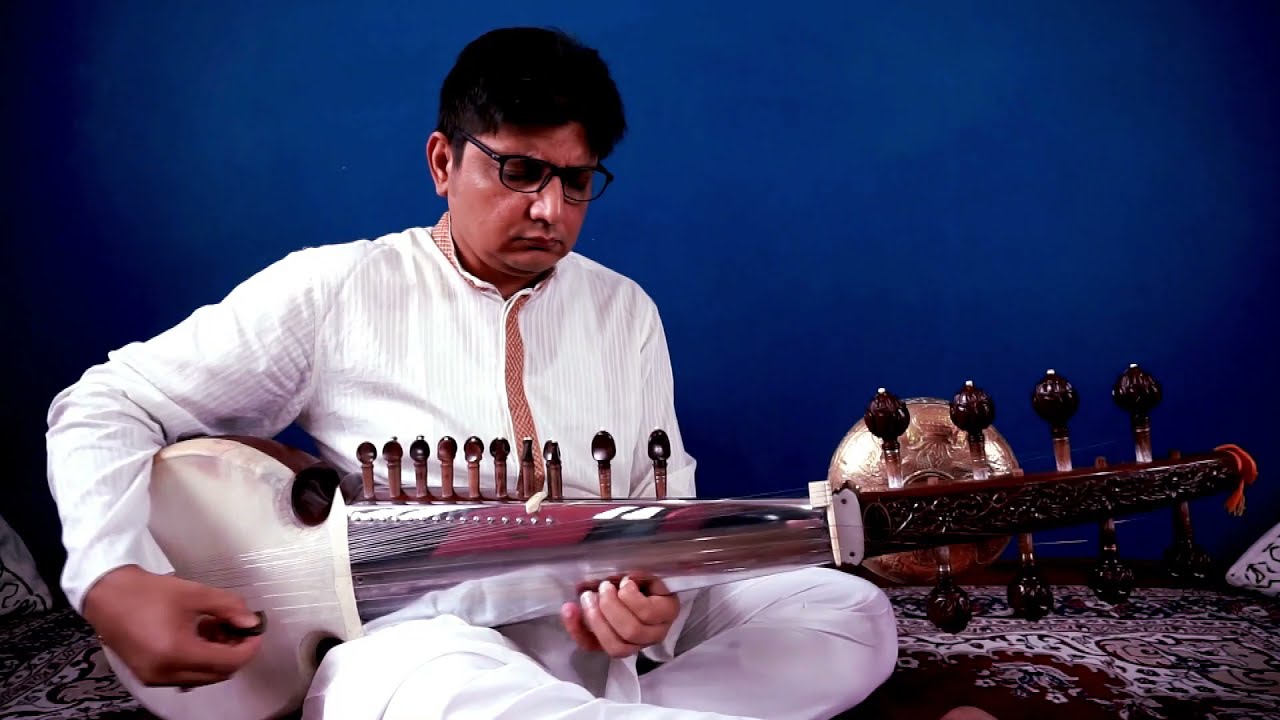In the image, a serious-looking man of Indian descent is depicted sitting cross-legged on a colorful, ornamental rug. He is playing a traditional Indian string instrument, likely a sarod, which has a long neck, rounded body, and numerous tuning pegs that resemble those of a guitar. The man's attire consists of a traditional white outfit, including white pants and a long-sleeved white top featuring a brown-collared jacket. He wears black glasses and has short dark hair. His focus is entirely on the instrument, as he looks down intently while strumming. Behind him, the wall is painted a deep blue, and a gold decorative object can be partially seen.